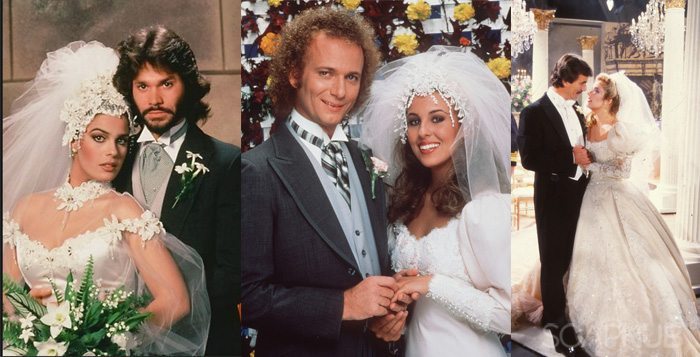The image is a collage of three distinct wedding-themed pictures, each featuring a bride and groom in various settings and poses. On the left, the couple stands side by side against a backdrop of brown tiles. The bride is elegantly dressed in a white gown, adorned with a veil, and holding a bouquet of white flowers with green leaves. The groom complements her in a tuxedo with a grey shirt, grey vest, and a floral decoration on his lapel. In the central image, another couple faces the camera, both smiling warmly. The groom is captured in the act of placing a ring on the bride's finger, with vibrant yellow flowers adorning the background. The bride mirrors the elegance of the first, in a white gown and veil, while the groom is dressed in a blue suit. Finally, on the right, a couple gazes into each other's eyes in an indoor setting replete with grand chandeliers and pillars. Both are dressed in traditional wedding attire; the groom in a black tuxedo, and the bride in a white gown and veil. This full-body shot contrasts with the upper torso focus of the other images, showcasing a more complete view of their outfits. Together, these three panels encapsulate the joy and elegance of wedding moments.